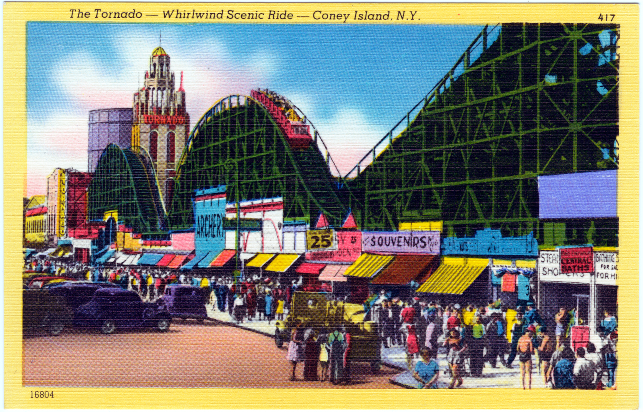The image depicts a vintage souvenir card illustrating the Tornado roller coaster at Coney Island, New York. The scene showcases a lively boardwalk with numerous concession stands, including an archery booth and souvenir shops, all bustling during the day. Towering behind the stands, the Tornado roller coaster, structured with prominent green metal bars, ascends and descends dramatically, culminating in a steep climb towards the top right corner of the image. The roller coaster itself features pink cars. To the left, near the bottom left corner, there are three or four purple vintage cars, likely from the 1950s, adding to the nostalgic ambiance of the scene. The illustration is bordered in yellow, with the text "The Tornado - Whirlwind Scenic Ride - Coney Island, New York" at the top. The numbers "417" and "16804" are printed in the upper right and bottom left corners, respectively. Notably, items are still priced as low as 25 cents, emphasizing the old-time setting of this charming depiction.